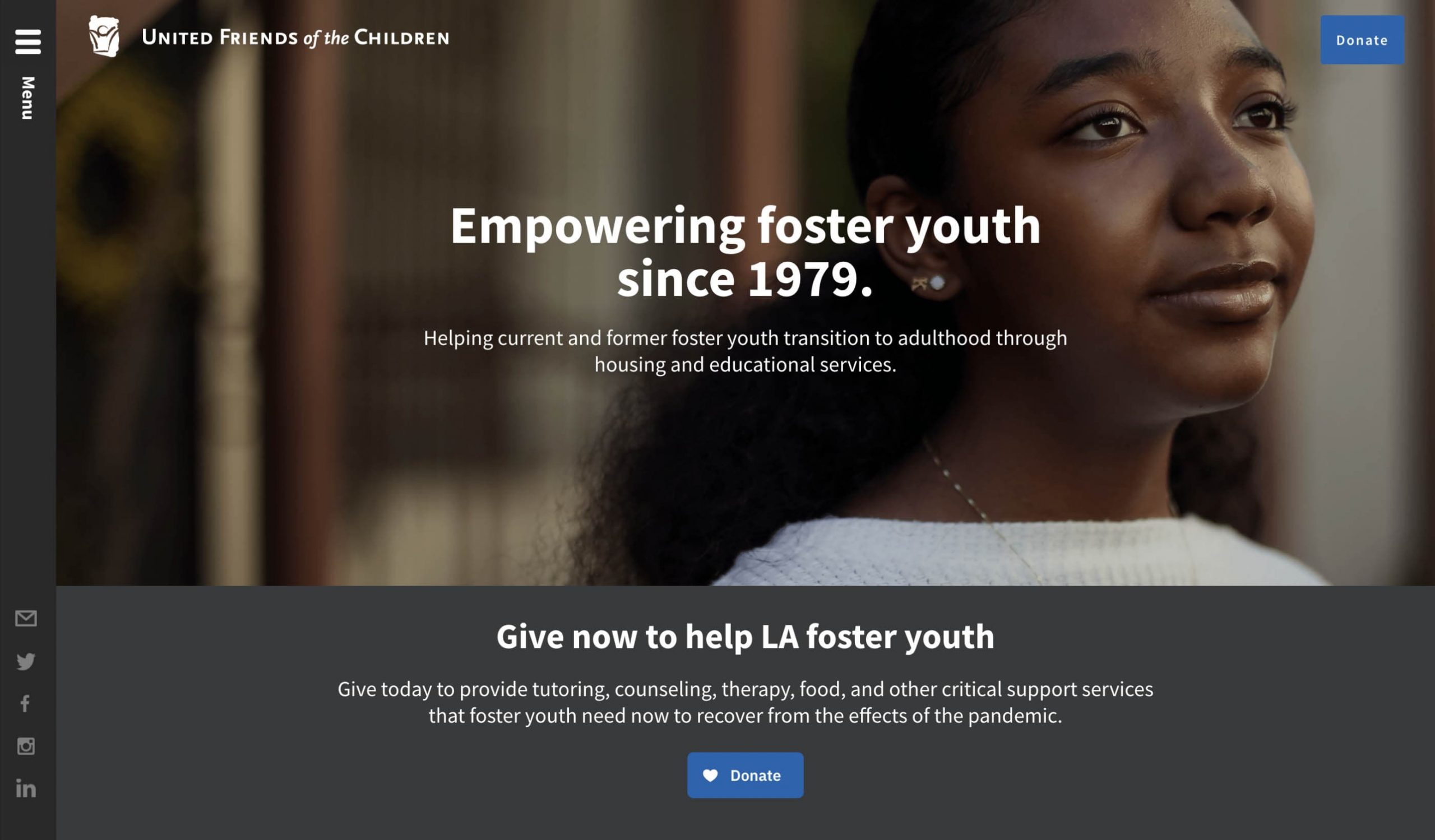The screenshot showcases a website for "United Friends of the Children." The top-left corner features the organization’s name, while the top-right corner prominently displays a blue "Donate" button. Central to the page, bold text reads "Empowering Foster Youth Since 1979." Directly beneath, a description elaborates: "Helping Current and Former Foster Youth Transition to Adulthood Through Housing and Educational Services."

Towards the bottom, a call-to-action headline states, "Given Out to Help L.A. Foster Youth," followed by a plea, "Give Today to Provide Tutoring, Counseling, Therapy, Food, and Other Critical Support Services that Foster Youth Need Now to Recover from the Effects of the Pandemic." Another blue "Donate" button, adorned with a small white heart on the left and the word "Donate" in white text at its center, is positioned just below the message. The background of the screenshot is a muted gray, emphasizing the text and buttons.